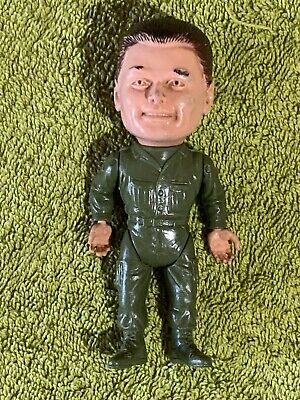This photograph captures an up-close view of a small plastic male action figure with a disproportionately large head and a smaller body. The action figure, dressed in an olive green army-like suit, is laying on its back on a light green, carpet-like background. The suit covers the figure entirely from head to toe, including dark green boots that blend into the outfit. The doll's face is characterized by a wide, smiling expression with small, dark brown or black eyebrows and a short brown, slicked-back hairstyle. The figure features poseable arms and legs that extend from the olive green outfit, showing light tan hands capable of holding objects. The background, resembling a towel or rug, provides a lime-green contrast to the darker green uniform, enhancing the figure's detailed appearance, which includes molded plastic buttons, pockets, and seams on the clothing.